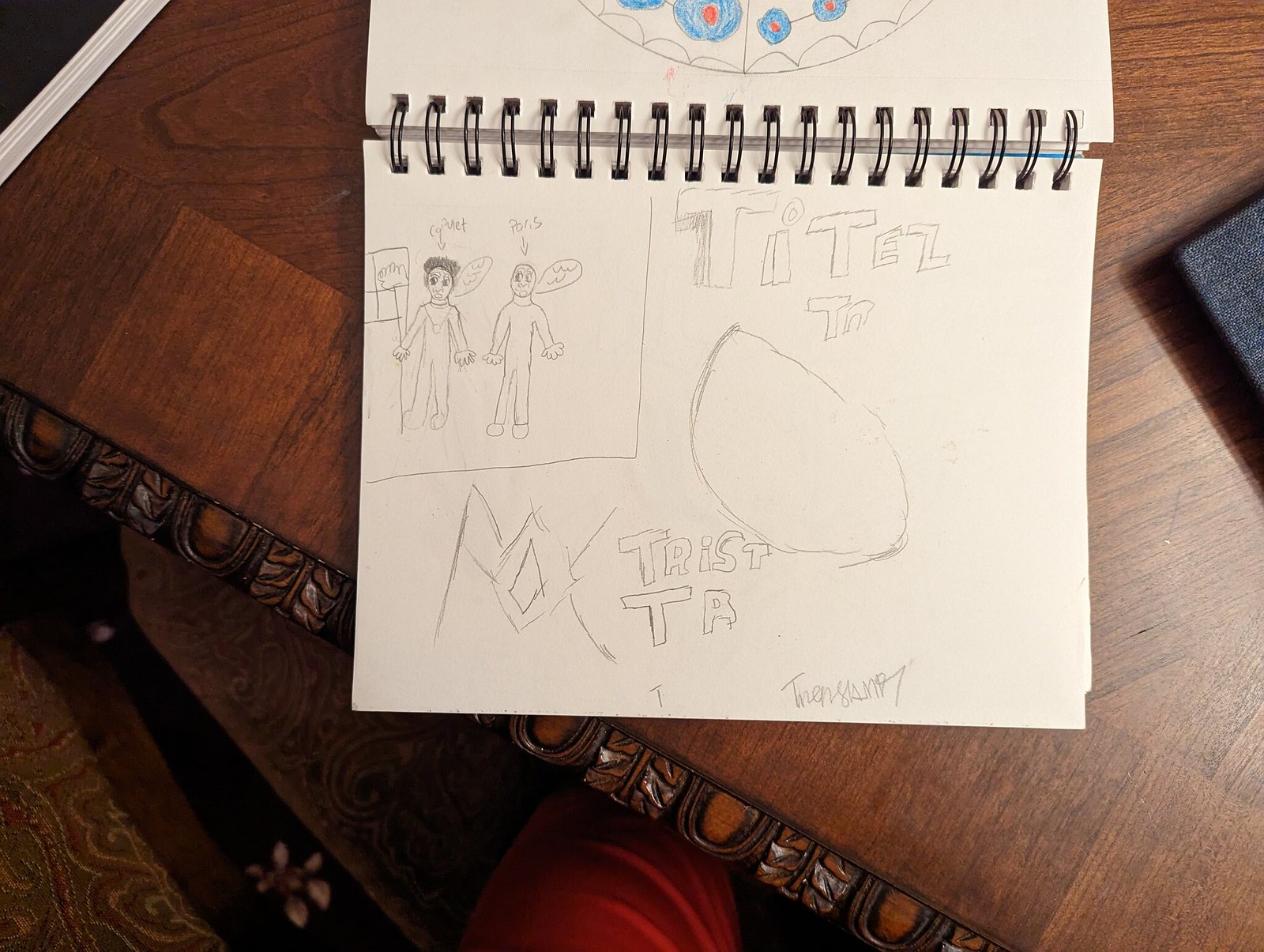A sketchbook lies open on a brown wooden table, displaying white pages filled with various pencil markings and illustrations. On the left page, scribbled words can be partially deciphered, such as "tell" and "Trist T R T A," along with cursive writing. Below the text, a half-circle shape is visible. This page also features a box containing a simple drawing of two people conversing beside a sign; one person has hair while the other appears bald. 

The right page of the sketchbook reveals a portion of a circular design with blue balls and red centers. Surrounding the sketchbook, there are other items placed on the table. To the right, a black object is seen, and in the top left corner, there appears to be another book with a black cover, revealing white pages in between. At the bottom of the image, an orange fabric, possibly a chair or someone's pants leg, is slightly visible, providing a hint of the surrounding environment.